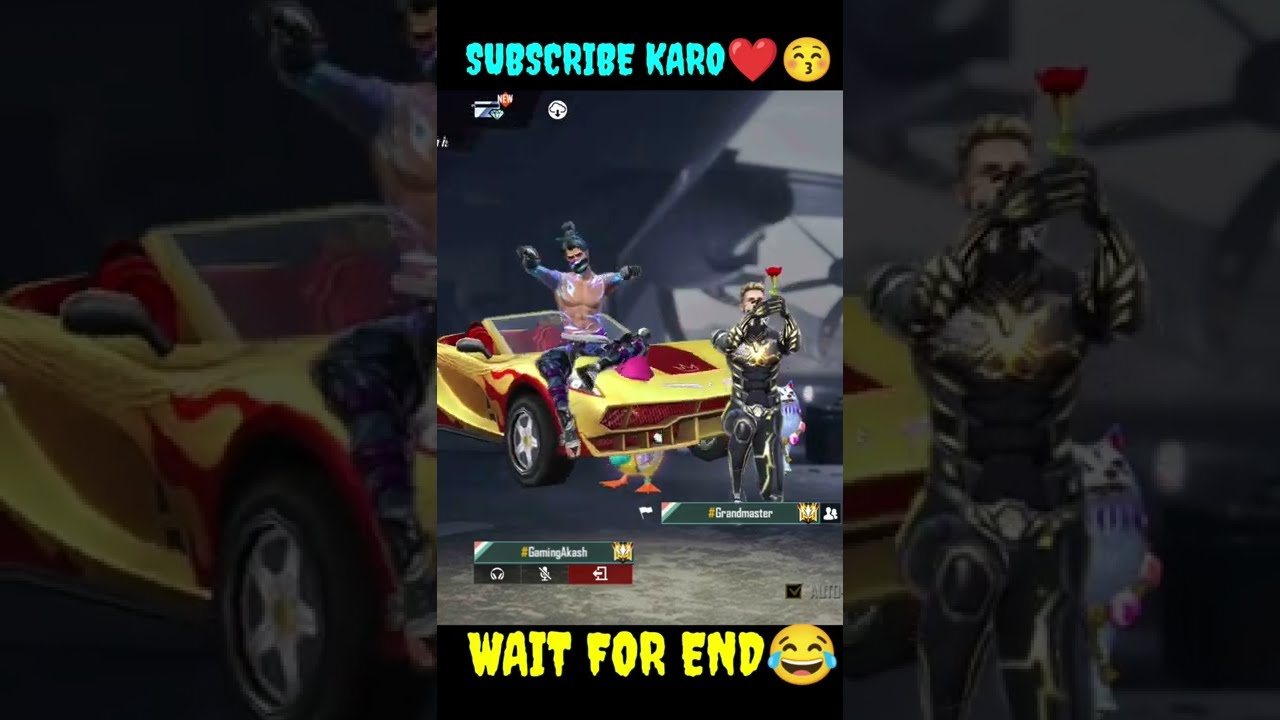The image is a horizontal rectangular screenshot from a video game, divided into three vertical sections. The central section features a red and yellow convertible car with two male characters: one shirtless character with black hair and dark patterned pants sitting on top of the car, and another character in silver armor with gold on the chest standing in front of the car, holding what appears to be a golden stick with a red top, possibly a flower. Above the central scene, within a horizontal black strip, the text "SUBSCRIBE KARO" in light blue capital letters is accompanied by a heart and kissing emoji. Below the scene, within another black strip, the text "WAIT FOR END" in yellow capital letters is followed by a laughing-crying emoji. The left and right sections are darkened close-up views of the central section: the left shows the red and yellow car with the shirtless man sitting on top, while the right focuses on the armored man holding the flower. Additionally, the text on the central image mentions "Grandmaster and Gaming Akash."